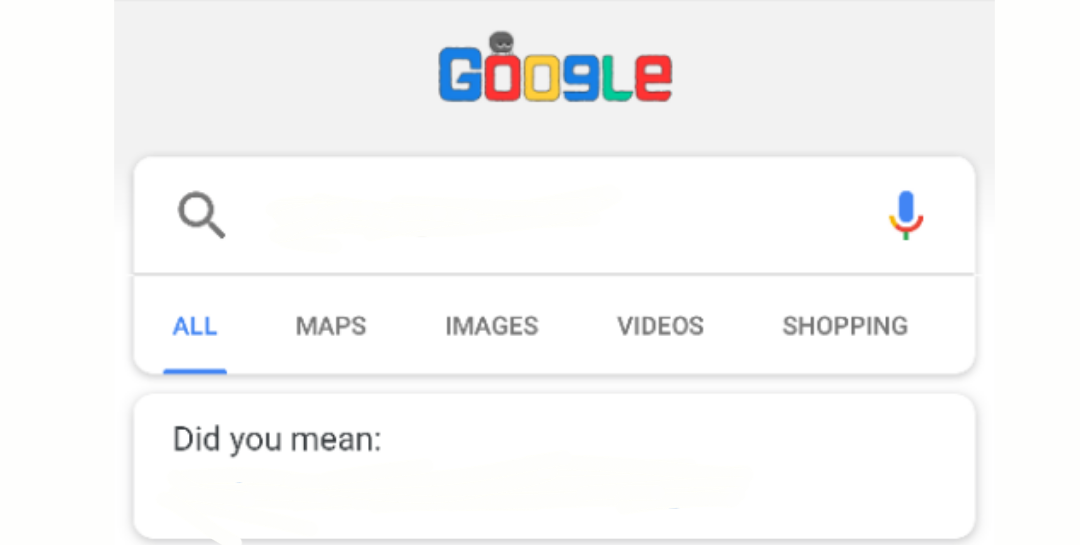The image is a landscape-oriented screenshot divided into two main sections. 

**Upper Section:**
- Background: Light gray
- Center: A unique Google logo with playful variations. 
  - The first letter "G" is in blue.
  - The first "o" is red with an overlay resembling a small bug, featuring a gray circle with dark black dots as eyes and white lines underneath, enhancing the bug-like appearance.
  - The second "o" is yellow. 
  - The second "G" is stylized to resemble the number nine.
  - The "L" is in green.
  - The "e" is in its usual small size.

- Beneath the Google logo is a search bar where the search icon is positioned on the left and a microphone icon on the right.

**Middle Section:**
- A thin, gray dividing line separates the sections.
- The header menu includes options labeled "All," "Maps," "Images," "Videos," and "Shopping." 
  - The "All" option is highlighted in blue and capitalized.

**Lower Section:**
- Begins with a white space, containing a large input form.
  - Text: "Did you mean:" followed by a colon, suggesting an alternate search suggestion for the user.

This detailed breakdown reflects a standard yet creatively altered Google search page, emphasizing the unique design elements of the logo and layout.